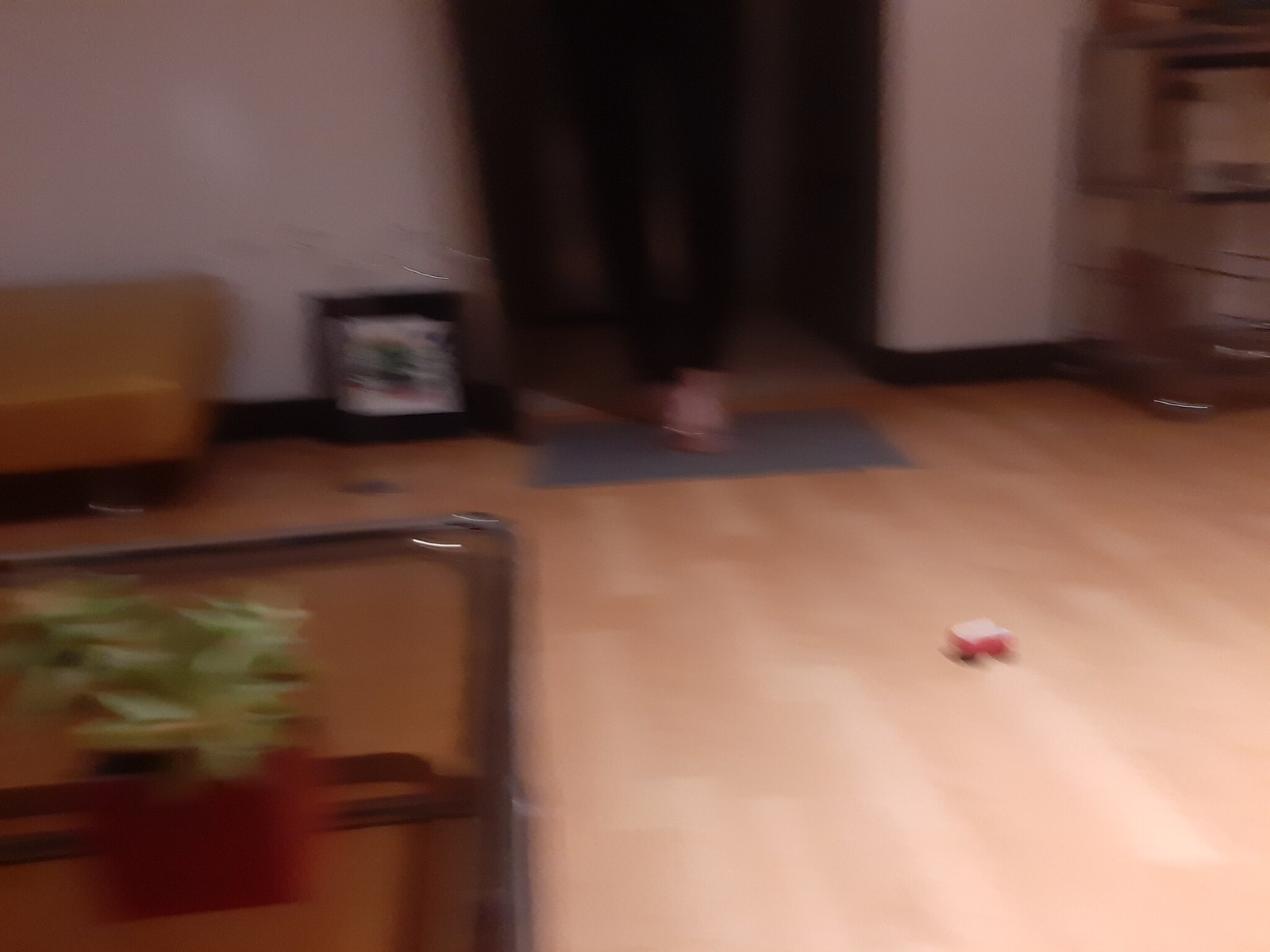In this dimly lit and highly out-of-focus indoor photograph, we observe a scene centered on a light tan hardwood floor that is slightly larger than it is tall. The lower left quadrant predominantly features a glass coffee table, identifiable by its metal rim and supporting legs. Atop this table rests a medium red planter housing a green plant, possibly adorned with a few indistinct white flowers. Adjacent to the table, the floor extends in a light wood tone and meets a white-walled background starting approximately 60% up the image.

In the upper portion of the image, there is a doorway through which only the thin black-clad legs of a person can be discerned. To the immediate left of this doorway stands a framed picture against the wall, while further left, a small ottoman draped in brown leather is visible. A gray rug lies in front of the doorway with an indeterminate object on it due to the blurriness. Meanwhile, the lower right quadrant contains a conspicuous wire shelf or kennel stack, positioned against the white wall with a distinct black trim.

Adding to the overall clutter, another object, potentially a toy, lies on the floor slightly right of center. Though no text is present in the image, the scene is interspersed with various elements rendered almost indistinguishable due to graininess and poor focus.